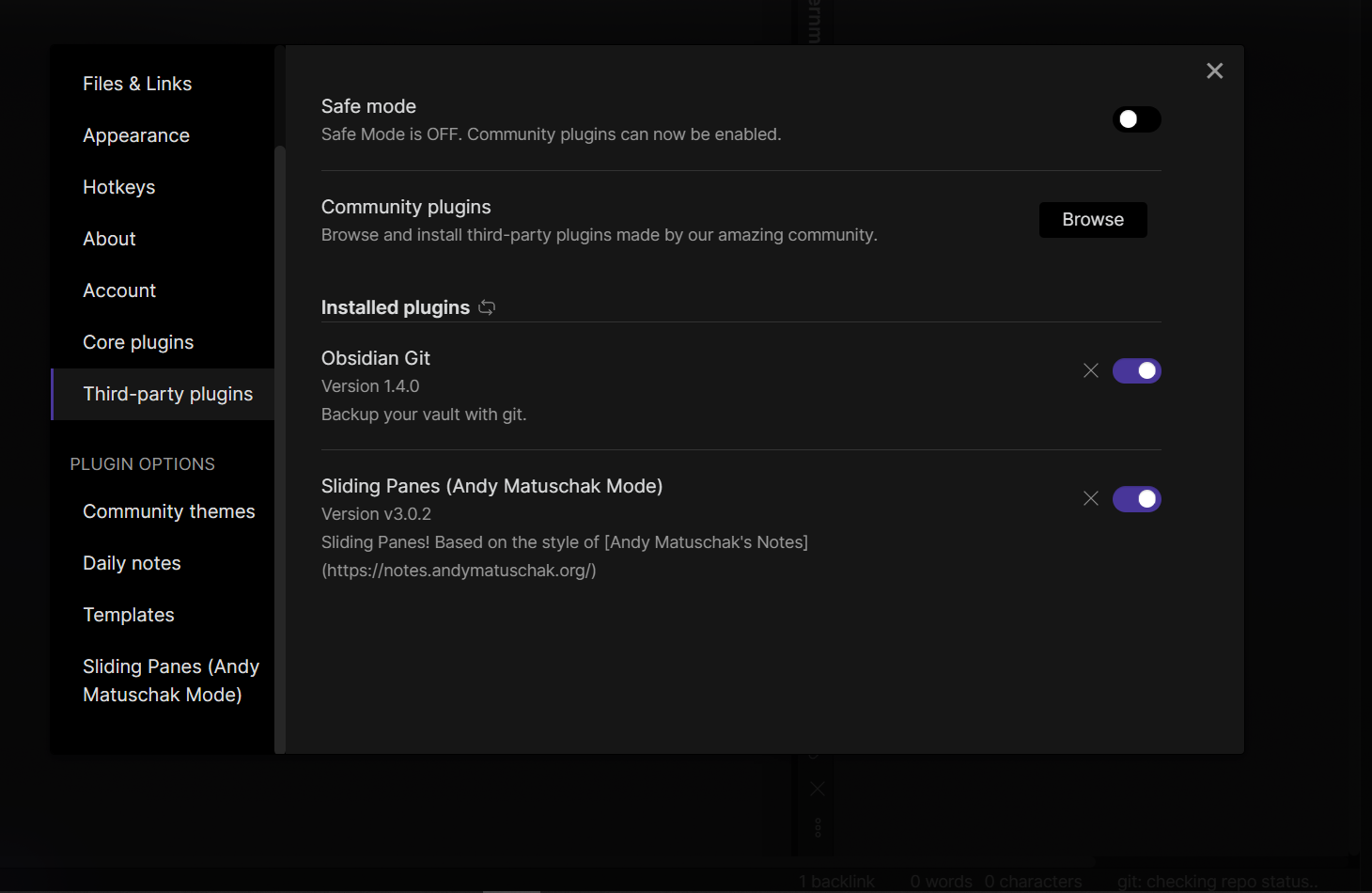In the image, a user interface for configuring a blogging or application platform is displayed. The background is a dark gray, overlaid with a darker vertical menu on the left side featuring white text labels including "Files and Links," "Appearance," "Hotkeys," "About," "Account," "Core Plugins," and "Third-Party Plugins," which is currently selected and highlighted with a lighter gray background.

Adjacent to this menu, the main panel provides detailed options for third-party plugins. At the top of this panel, it reads "Safe Mode," "Community Plugins," "Installed Plugins," and "Sliding Panes." The "Safe Mode" is turned off. Under "Community Plugins," there's a button labeled "Browse" on the right. The "Installed Plugins" section lists "Obsidian Git version 1.4.0," described as a tool to back up your vault with Git, and it shows a toggle switch in the "On" position with a purple indicator.

Below this, there's another entry for "Sliding Panes," labeled as "Sliding Panes by any metachasic mode," version 3.0.2. This plugin is based on the style of NWB2CASQ's notes and includes a toggle switch in the "On" position with a purple indicator. A link to NWB2CASQ's website is provided directly beneath this description.